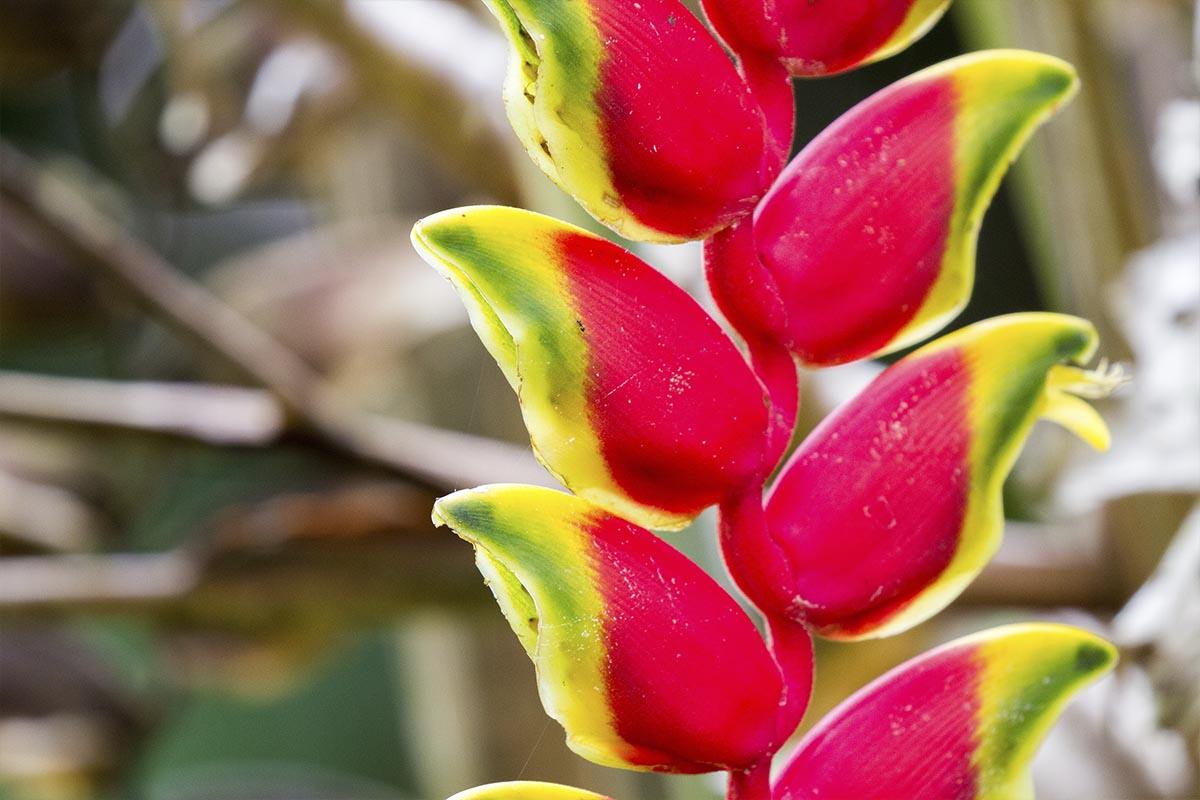This vibrant, close-up photograph captures a striking Heliconia plant, prominently featured against a blurred backdrop of brown foliage and indistinct jungle greenery. The photo, taken in landscape orientation, places the Heliconia slightly off-center to the right, emphasizing its unique structure. The plant boasts a curving red stalk that sinuously snakes down the image in an S-shaped pattern, with flowers dangling alternately on either side, resembling a natural ladder. Each flower is substantial, bearing a teardrop or talon shape with a fat and bulbous appearance. Their vivid coloration includes a split design: one half showcases a bright red hue transitioning to the other half in vivid yellow, accented with touches of black along the pointed tips. A few green streaks are also visible, adding to the plant's tropical allure. This detailed depiction highlights the Heliconia's exotic beauty and intricate design, making it the focal point of the photograph.